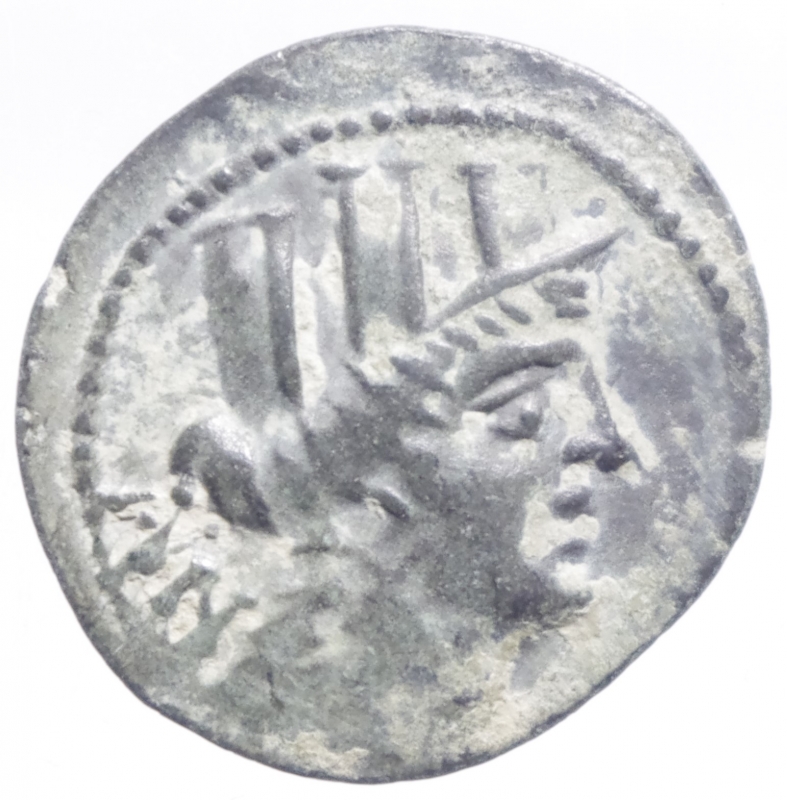The image features an ancient coin-like object that is roughly circular and appears asymmetrical. The material of the object seems to be stone, depicted in a gray hue with patches of white powder on the surface, giving it an aged and worn appearance. The edges are rough and chipped, adding to its antiquated look. The coin's centerpiece is an engraved human face, staring towards the right. Surrounding the top of the face is a pattern resembling a ring of dots or a decorative border. The figure appears to be wearing a crown or hat with vertical lines, indicative of a possible historical or iconic significance. The background of the image is white, and the base of the neck of the profile is somewhat blurred, masking further detail. The overall profile bears a resemblance to the Statue of Liberty, characterized by a prominent nose and a regal demeanor.